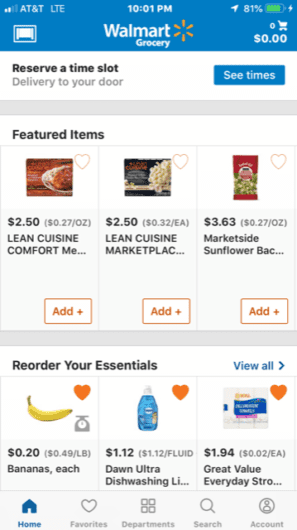The image displays a smartphone screen showing the Walmart grocery delivery page. At the top of the screen, the status bar indicates "AT&T LTE," the time "10:01 PM," the battery level as "81%," and a battery icon.

Centered below, the screen displays the Walmart logo with the word "Grocery." Directly under this, there is an icon of a shopping cart with "$0.00" next to it. The text below reads "Reserve a time slot" and "Delivery to your door," followed by a button labeled "See times."

Further down, the section titled "Featured items" showcases thumbnails of grocery products. Despite the images being somewhat blurry, the descriptions are legible. On the left, there is a food item priced at "$2.50" with "27 cents an ounce," identified as "Lean Cuisine Comfort." To its right is another Lean Cuisine product, labeled "Lean Cuisine Marketplace," priced at "$2.50" and "32 cents each." Next to these is a red bag labeled "Market Side Sunflower," priced at "$3.63" and "27 cents an ounce." Each item has an "Add" button with a plus sign next to it.

The section below these items is titled "Reorder your essentials," featuring images of frequently purchased items: a banana, a bottle of Dawn dish soap, and a package of bath tissue, each with a heart icon beside them. Specifically, the banana is listed at "20 cents," with a note of "49 cents a pound." The Dawn Ultra Dishwashing soap is priced at "$1.12," with the unit price "$1.12/fluid ounce." The Great Value bath tissue is labeled "$1.94," with "2 cents each" as the unit price.